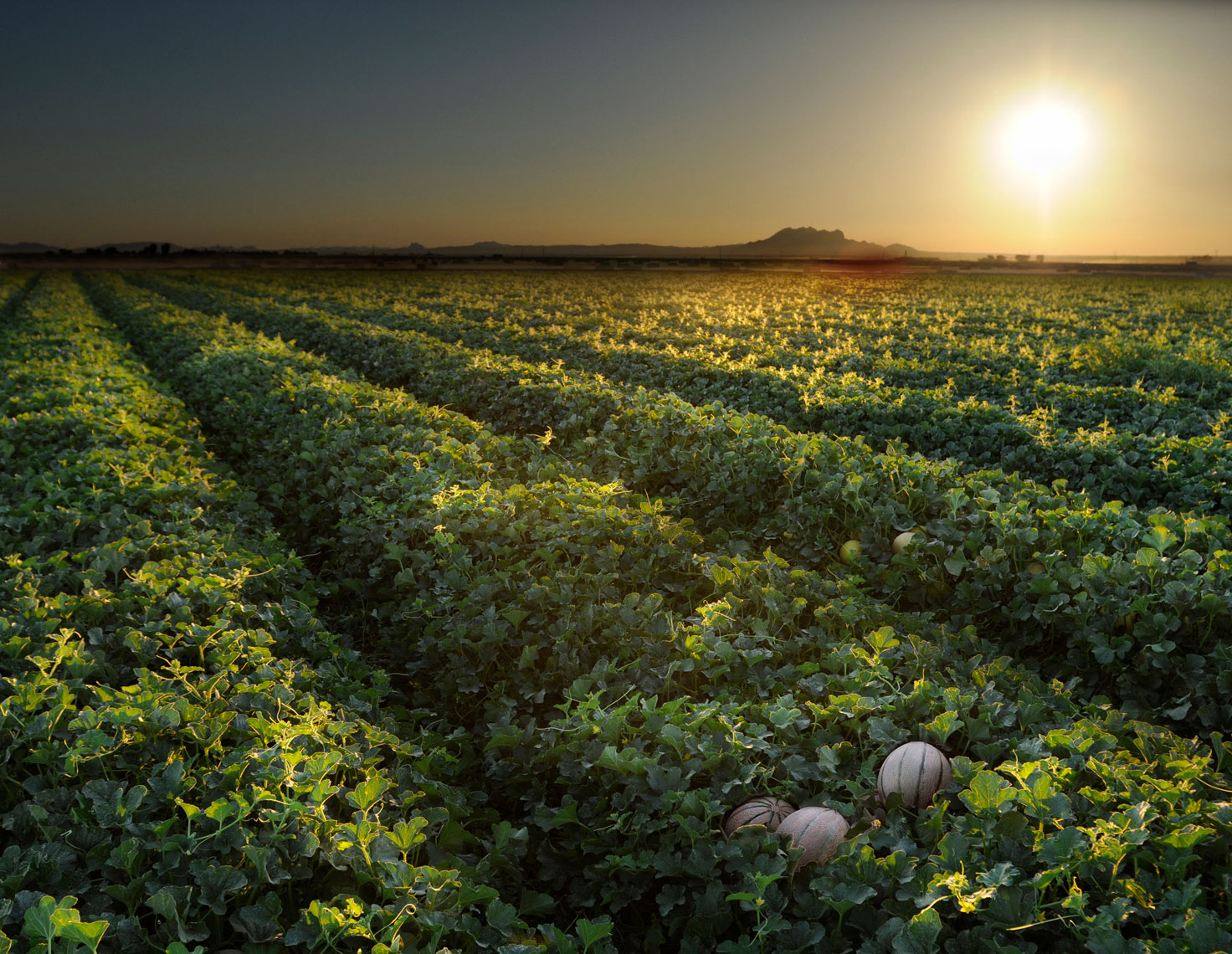This photograph captures a vast agricultural landscape during what appears to be either sunset or sunrise, with the sun brimming just above the horizon, casting a golden hue over the scene. The sky above is clear, with the sunlight illuminating the tops of the leaves, creating a striking contrast against the deepening shadows. In the foreground, rows upon rows of lush green crops stretch out into the distance. Among the crops, numerous round, striped vegetables—likely watermelons or possibly squash—are distinctly visible, lending a sense of abundance to the field. The expansive field is meticulously organized into neat rows, evoking an industrial-scale farming operation. In the background, the faint outline of a mountain range emerges against the bright sky, suggesting a locale that could be reminiscent of the agricultural valleys of California or the arid regions near Arizona or Nevada. The juxtaposition of the lush, green foreground with the more barren, shadowed expanse in the background highlights the complex and varied landscape of the area.